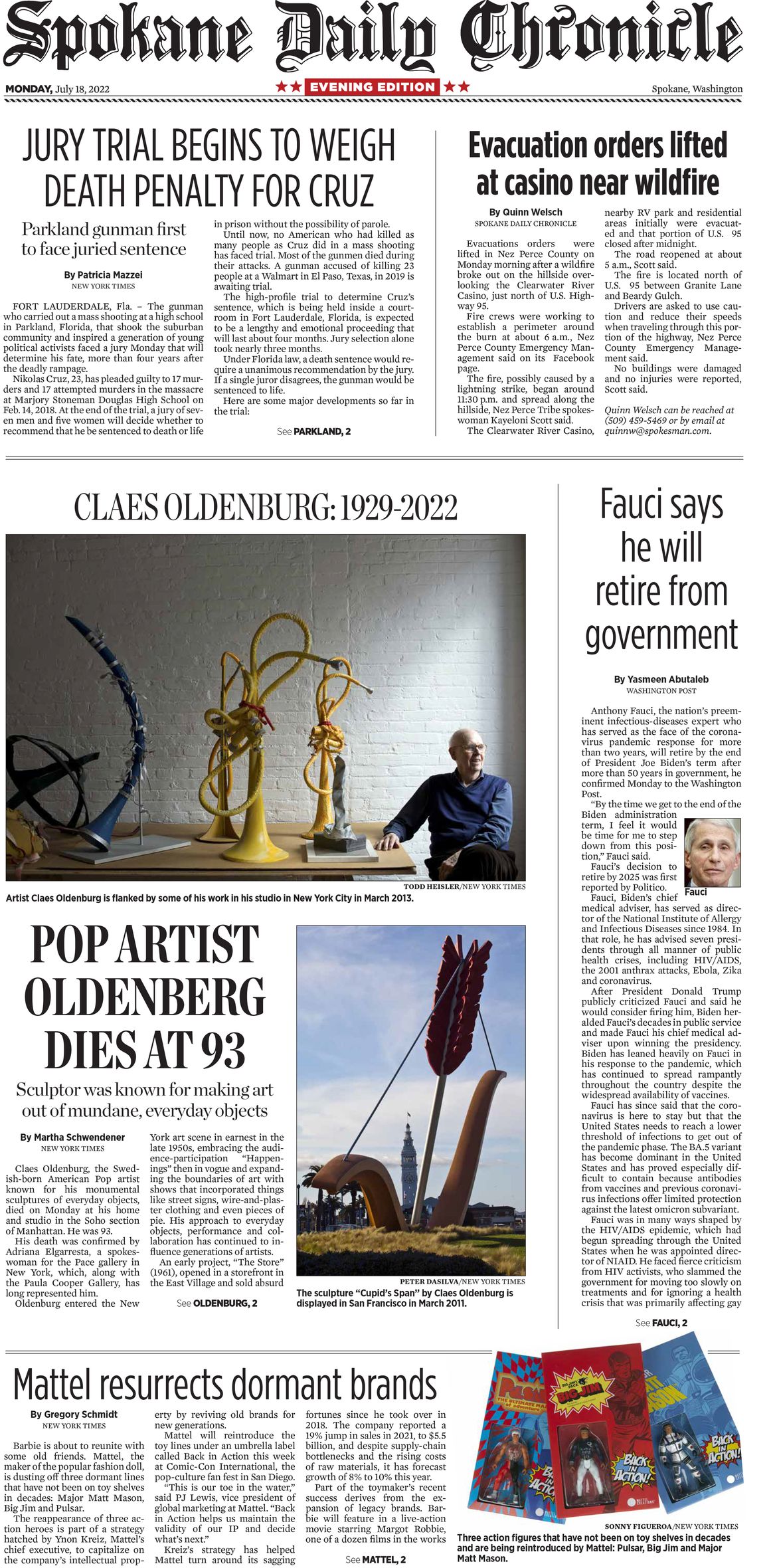Screenshot of the front page of the Spokane Daily Chronicle, Edition 9: The central heading announces "Jury Trial Begins to Await Death Penalty for Cruz." On the top right, another headline states "Evacuation Orders Lifted at Casino Near Wildfire." Beneath this, an obituary headline reads, "Kales Oldenburg, 1929-2022," followed by "Pop Artist Oldenburg Dies at 93." To the left, another article is titled "Mattel Resurrects Dormant Brands," and on the bottom right, a headline announces "Fossey Says He Will Retire from Government." This detailed layout showcases a diverse range of current events and significant news stories featured in the newspaper.